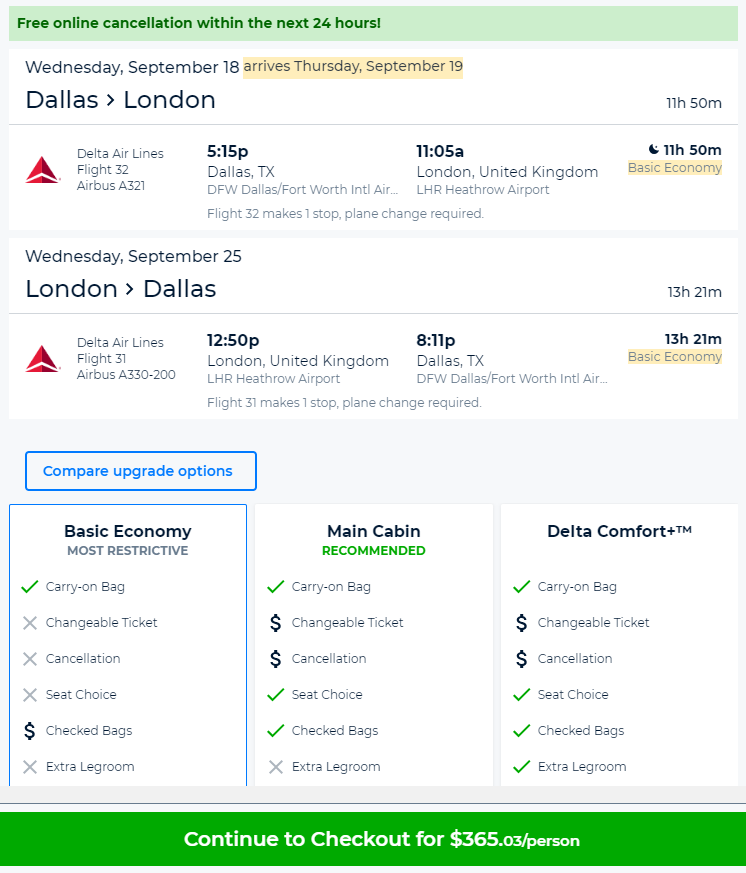A screenshot from a tablet displays flight options for a trip between Dallas, Texas, and London, United Kingdom, via Delta Airlines. The top banner highlights a policy of free online cancellation within the next 24 hours. 

The outbound flight, scheduled for Wednesday, September 18th, and arriving on Thursday, September 19th, spans 11 hours and 50 minutes. The return journey departs London on Wednesday, September 25th, lasting 13 hours and 21 minutes back to Dallas. 

The seating option for this itinerary defaults to Basic Economy, which includes only a carry-on bag. Below, there's a comparison of upgrade options such as Main Cabin, which allows changeable tickets, cancellations, seat choices, and checked bags, and Delta Comfort, which offers all Main Cabin benefits plus extra legroom.

At the bottom of the screen, a green bar with white text prompts users to "Continue to Checkout" for $365.03 per person.